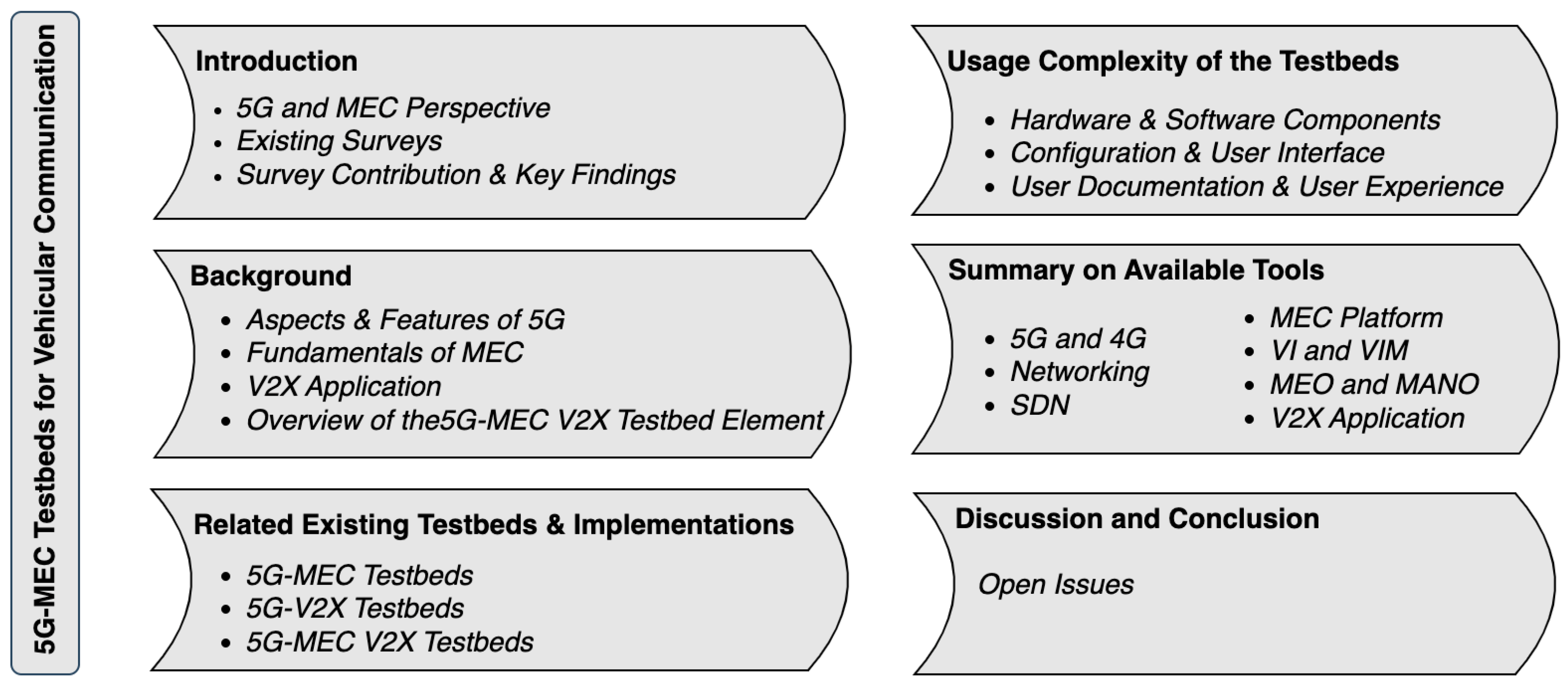The image displays a structured outline divided into grey tabs, set against a white background with pale lilac accents. Along the left side is a vertical box with "5G-MEC Testbeds for Vehicular Communication" written from bottom to top. The outline starts with an "Introduction" tab, detailing the 5G and MEC perspectives, existing surveys, and survey contributions and key findings. Following this is the "Background" tab, which includes aspects and features of 5G, fundamentals of MEC, the V2X application, and an overview of the 5G-MEC V2X testbed elements. Next, "Related Existing Testbeds and Implementations" is broken into three sections. Moving on, the "Usage Complexity of the Testbeds" tab highlights three bullet points. "Summary on Available Tools" is detailed under seven bullet points. The final tab, "Discussion and Conclusion," lists open issues. The chart presents this information in a visually distinct manner, using a thick arrow motif for organization, making it easy to follow and comprehend.